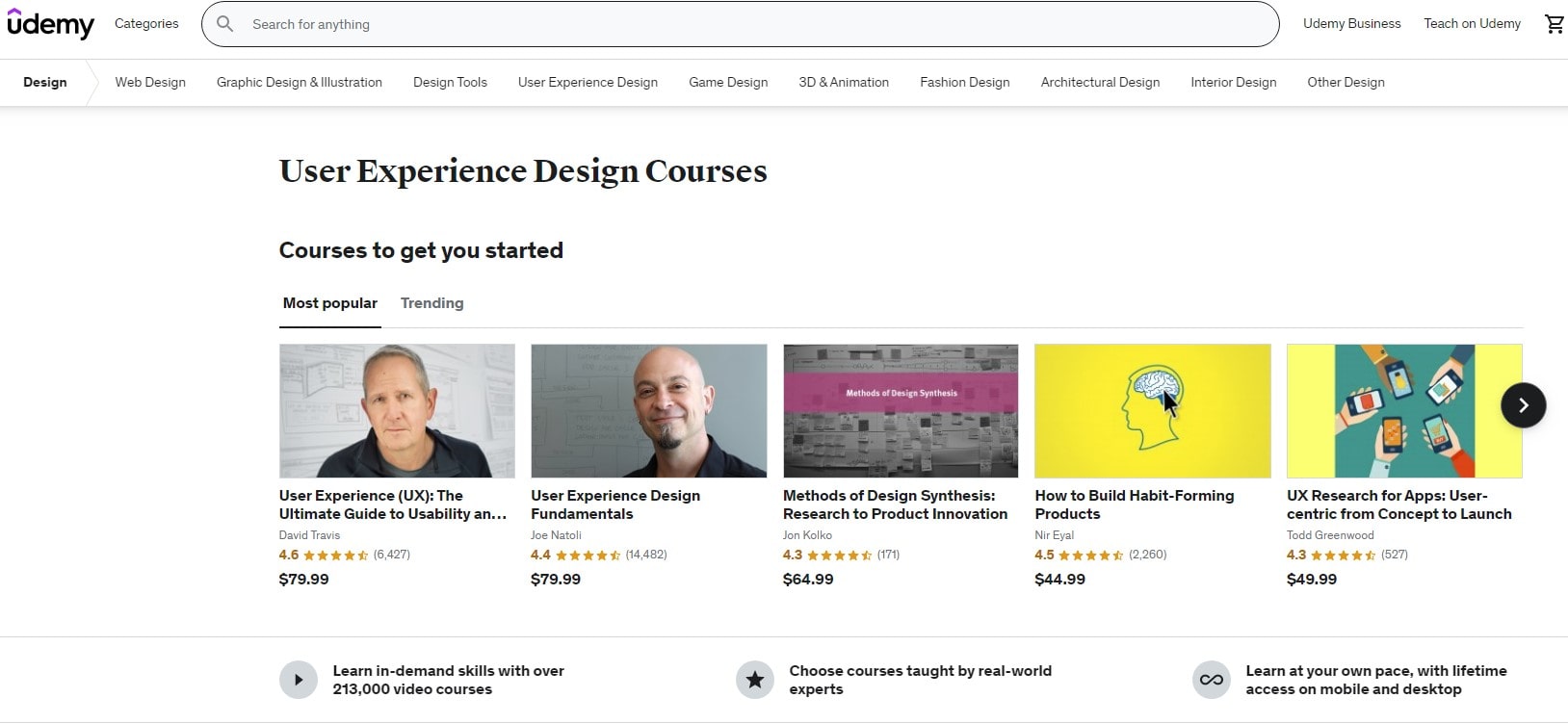The screenshot is taken from the Udemy website, prominently featuring its distinctive logo at the top left corner, characterized by the lowercase "udemy" text in black, with a unique purple accent mark resembling a small upward arrow (caret) placed above the "u". Adjacent to the logo is the "Categories" tab, followed by an elongated, capsule-shaped search bar reading "Search for anything," which spans the width of the interface.

Further to the right, the menu extends with options such as "Udemy Business," "Teach on Udemy," and a shopping cart icon for users' convenience. 

A detailed navigation menu unfolds, listing various design disciplines: "Design," "Web Design," "Graphic Design & Illustration," "Design Tools," "User Experience Design," "Game Design," "3D & Animation," "Fashion Design," "Architectural Design," "Interior Design," and "Other Design." 

Beneath this menu, the section is titled "User Experience Design Courses," offering curated segments like "Courses to Get You Started," "Most Popular," and "Trending." Below, individual courses are displayed with their respective thumbnails, titles, ratings, and prices:

1. **User Experience (UX): The Ultimate Guide to Usability**  
   - Rating: 4.6 out of 5  
   - Price: $79.99  

2. **User Experience Design Fundamentals**  
   - Rating: 4.4 out of 5  
   - Price: $79.99  

3. **Methods of Design Synthesis: Research to Product Innovation**  
   - Rating: 4.3 out of 5  
   - Price: $64.99  

4. **How to Build Habit-Forming Products**  
   - Rating: 4.5 out of 5  
   - Price: $44.99  

5. **UX Research for Apps: User-Centric from Concept to Launch**  
   - Rating: 4.3 out of 5  
   - Price: $49.99  

At the bottom of the image, three key selling points are highlighted:
- Access over 213,000 video courses to learn in-demand skills.
- Choose from courses taught by real-world experts.
- Enjoy the flexibility of learning at your own pace with lifetime access on both mobile and desktop platforms.